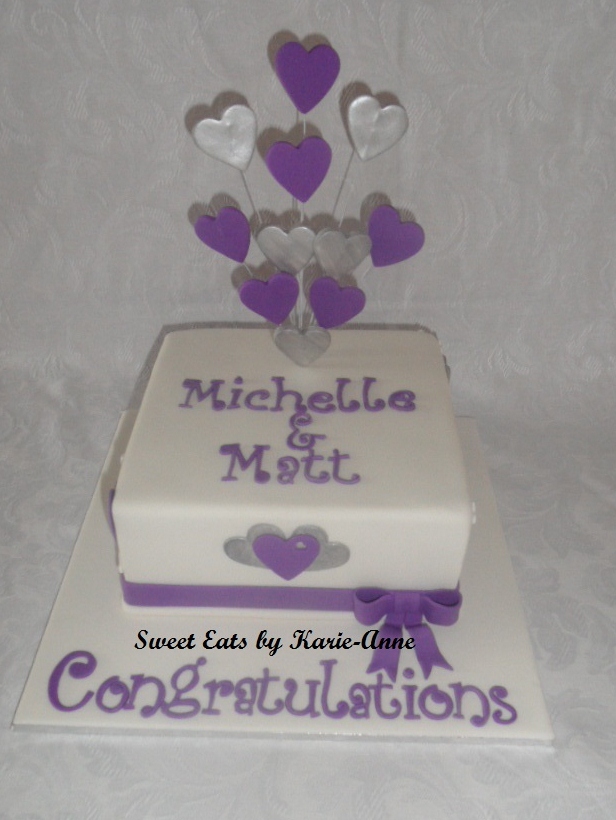This photo features an elegantly decorated square wedding cake placed against a mottled gray and white tablecloth background. The cake, adorned with smooth white fondant, prominently displays the names "Michelle & Matt" written in purple, with decorative dots accentuating each letter. A purple heart is centered on the front side of the cake, flanked by two smaller silver hearts. A tasteful purple fondant ribbon encircles the base, creating a coordinated look with a purple rectangular stripe and a bow at the lower front edge. Beneath the cake, on its white display board, the word "Congratulations" is scripted in a swirling purple font. Adding a whimsical touch, a topper featuring a spray of silver and purple hearts on thin posts gracefully extends above the cake, further enhancing the celebratory design. The bottom rim also highlights the phrase "Sweet Eats by Carrie Ann" in black, underscoring the cake’s custom craftsmanship.